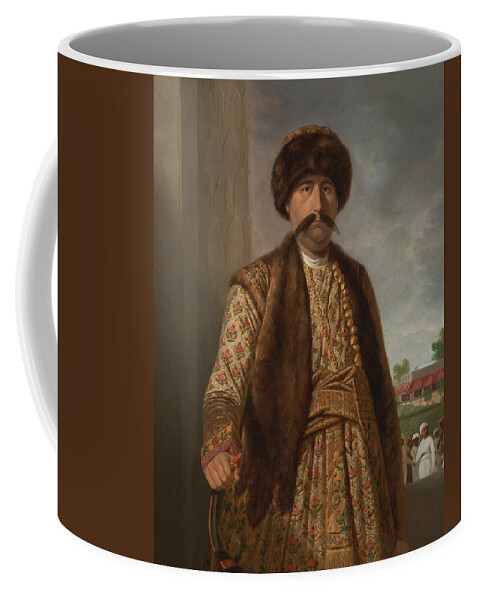This image depicts a digitally-rendered, large coffee mug set against a plain white backdrop, appearing as a prototype design likely created on a custom product site. The mug’s handle and interior are solid white, while the exterior showcases an intricate scene reminiscent of a 16th or 17th-century painting. In the foreground, a stern-looking male figure, evocative of a Turkish or Eastern European nobleman, commands attention. He dons a fur hat akin to a Russian turban, a pointed mustache extending past his face, and an ornate bronze and brown robe with intricate patterns and a beaded necklace, signifying his high status. His fur vest and grand attire further embellish his noble or warrior status. He holds a knife, adding to his formidable presence. The background unveils a vintage scene featuring men in white robes and caps amidst huts and houses with red roofs, likely situated in a Middle Eastern setting. The sky above shows dark clouds, contributing to the overall dramatic and historic ambiance of the mug’s design.